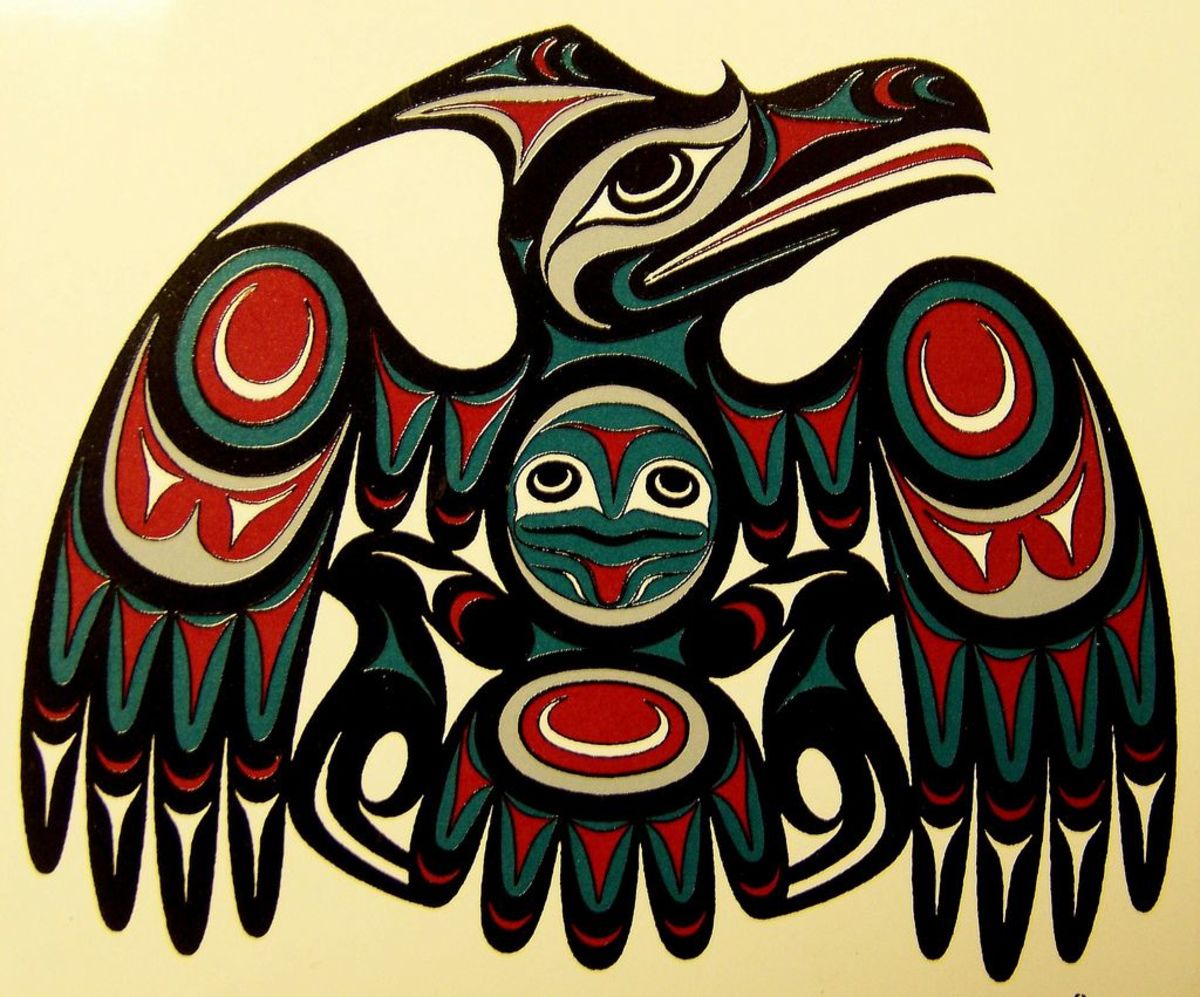This is a photograph of a stunning artwork reminiscent of Aztec design, depicting a striking bird. The bird is rendered in a rich palette of black, white, red, and teal. Its wings are exquisitely feathered—primarily black with a white center. Above the wings, red crescent shapes gracefully arc, adding a dynamic contrast. As your eye travels up the feathered wings, intricate patterns of red triangles and teal accents emerge, contributing to the artwork’s visual complexity.

The bird's head is adorned with red triangles and teal crescent shapes, and it features a vivid red tongue and a sharp black beak. A prominent, large white eye with a black center stands out strikingly in the center of the bird, situated between its wings and the collarbone area, giving the piece an almost mystical aura.

The abstract face of the bird is exceptionally detailed, featuring bold teal lips, eyes shaped like black and white crescent moons, a red triangular motif, and a vivid red tongue. Set against an ivory background, the artwork vividly captures the essence of ancient Aztec aesthetics while also infusing modern elements, resulting in a captivating and intricate visual experience.